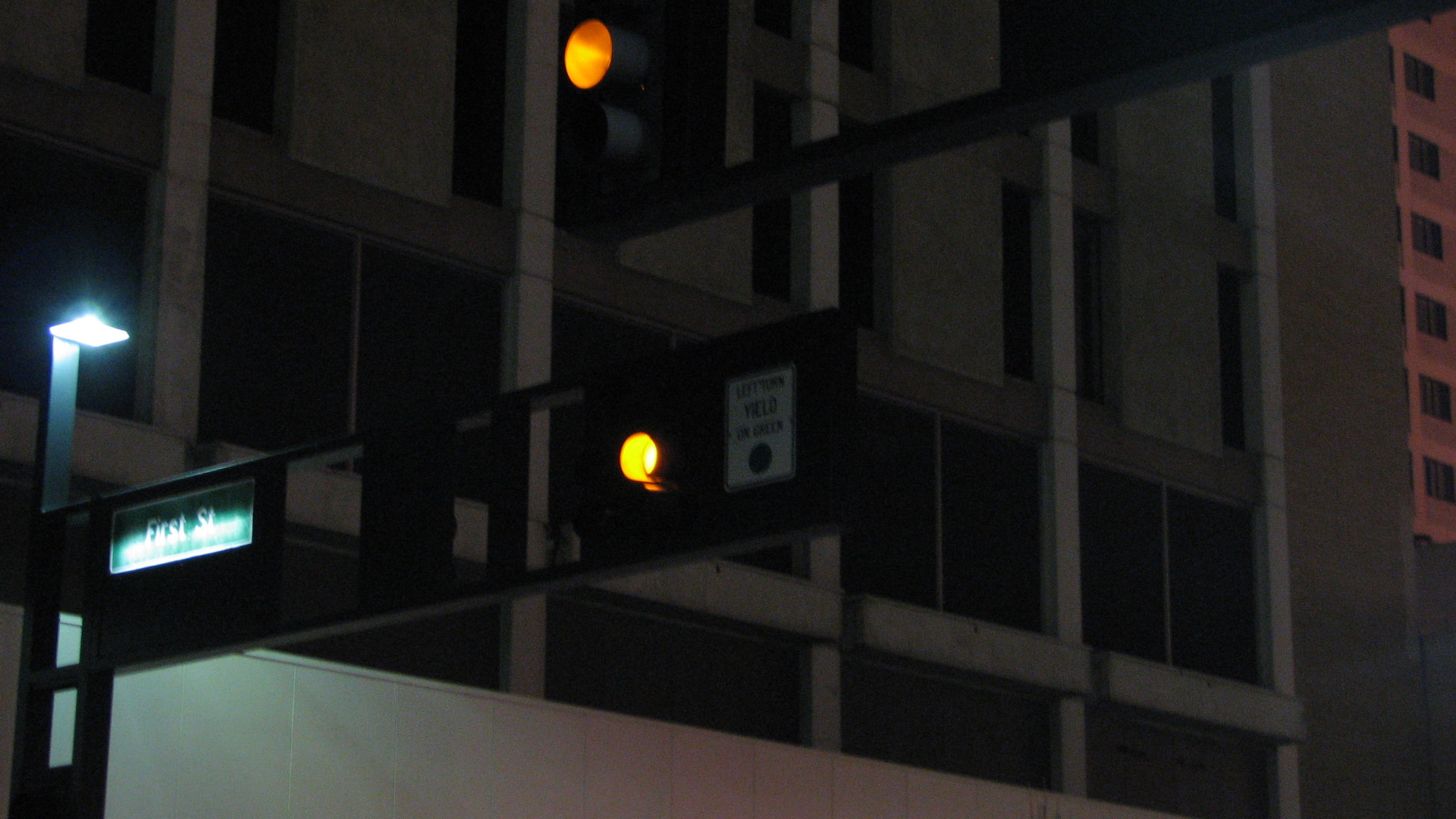A simple yet detailed photograph capturing a traffic intersection framed by an imposing concrete building with numerous windows in the background. The focal point is a pair of stoplights, one positioned above the other, both glowing yellow. A sign attached to the right side of the traffic light instructs drivers with the message, "Left Turn Yield on Green." To the left of the traffic light, a green street sign with white lettering indicates "First Street." Adjacent to this sign, a bright street lamp casts a glow that clearly illuminates the name of the street.